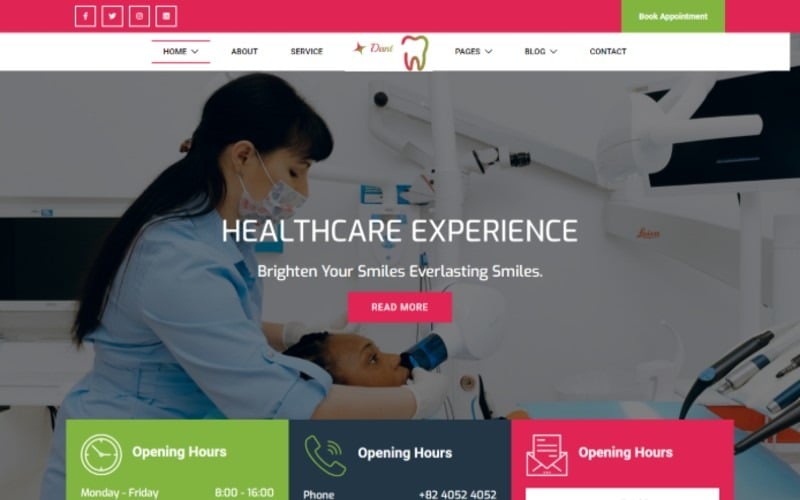The top section of this website features a red background with white-outlined squares representing various social media icons. The first icon displays the acronym for Facebook, the second one is a bird silhouette for Twitter, albeit slightly blurry. The next two icons are indistinguishable, but one appears to represent Instagram with a camera symbol, while the other could likely be LinkedIn. 

Beneath this, the red background continues, and there are two green rectangles with white text that read "Book Appointment." Adjacent to these, a navigation menu is set against a black background, with the "Home" tab highlighted by red lines above and below, indicating that the user is on the home page. Other tabs include "Services," "Blog," and "Contact."

The main image showcases a dentist with black hair pinned up by a brown hair clip, wearing a white, blue, and red face mask, and a blue button-down shirt with sleeves rolled up to three-quarters length. She is attending to a patient with brown skin, whose mouth is open. The dentist is wearing gloves and using a piece of white and blue equipment to examine the patient's mouth.

Above the image, a white text announces, "Healthcare Experience: Brighten Your Smiles, Everlasting Smiles." Below it, a red rectangle invites visitors to "Read More." At the bottom of the section, a green rectangle lists the opening hours in white text: "Monday to Friday, 8 a.m. to 4 p.m."